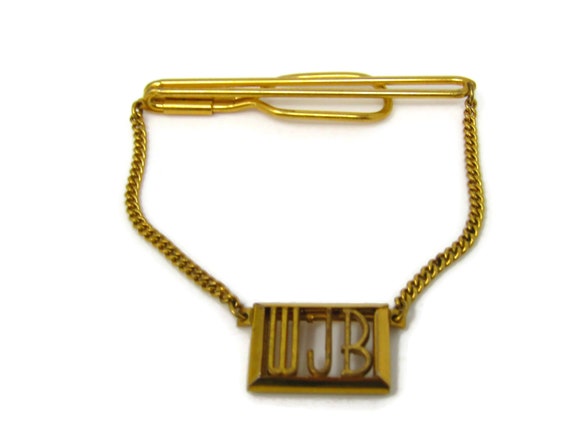This photograph showcases a piece of gold jewelry set against a white background, prominently featuring the initials "WJB" in the center. The jewelry piece, which could potentially be a necklace, tie clip, or bracelet, includes a square-shaped pendant where the initials are housed within an open, beveled gold frame. Two dense, short gold chains attach this pendant to a horizontal, tubular top section that likely includes a clasp mechanism. This piece appears to be distinctive and eye-catching, possibly assumed to be worn by a young adult or someone seeking to make a statement, rather than for everyday or professional attire. The clasp design suggests it secures around the back, offering a sturdy but possibly less comfortable fit.